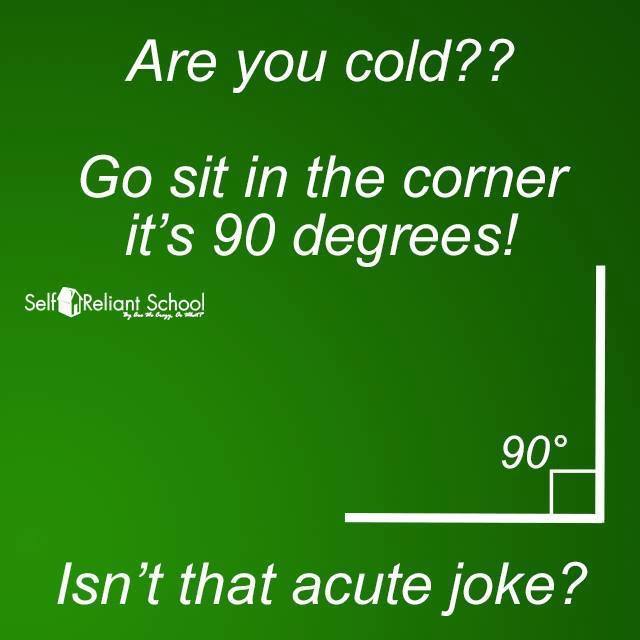The image appears to be a green poster resembling an advertisement or billboard. The background gradient transitions from a lighter green in the lower left to a darker green in the upper right. Dominating the poster are large white letters with the text aligned vertically. At the top, it reads "Are you cold??". Below that, with a gap in between, the text continues, "Go sit in the corner. It's 90 degrees!". Below this central message, there is a small logo depicting a little schoolhouse between the words "Self" and "Reliant School". In the lower right corner, a right angle illustration includes the text "90 degrees" within the angle. Beneath this, the poster concludes with the playful caption, "Isn't that a cute joke?"